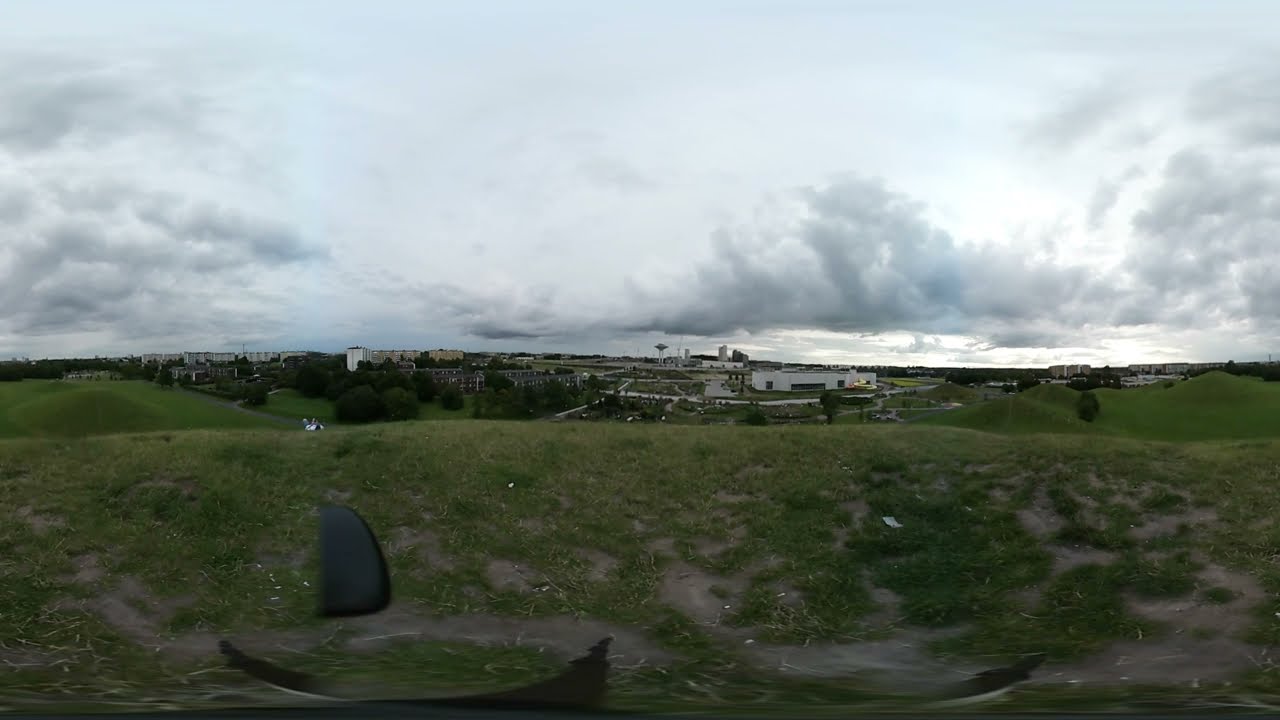The photograph depicts a vast, somewhat hilly grassy field, primarily covered in well-maintained short grass with occasional patches of dirt. Throughout the field, particularly on the left-hand side, there are a number of taller, round bushes. In the background, various buildings are visible, including some gray structures and a prominent white building more towards the center. The right-hand side features additional buildings and white walkways. The sky, occupying the upper half of the image, is pale blue and grayish with substantial cloud cover, making the scene appear somewhat dark as the sunlight struggles to break through. The presence of big clouds is noticeable on both the left and right sides of the image. Two black objects, possibly plastic, lie indistinctly in the foreground. The entire scene gives an impression of a cloudy day, with no people or text visible in the picture. The image may appear slightly warped, particularly towards the bottom, giving a sense of a 360-degree or VR capture.